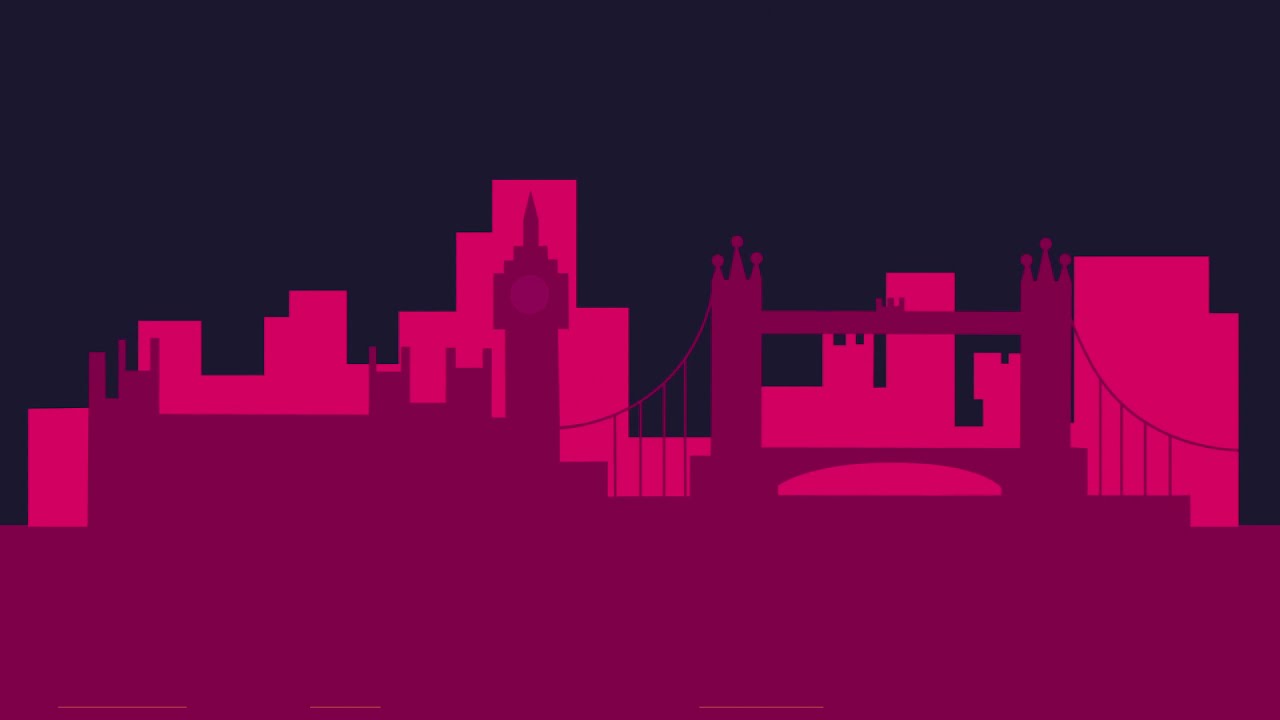The image appears to be a graphic, minimalist illustration of a cityscape at night, potentially depicting London. The scene is stark, with a black background setting off the vibrant city elements. The skyline features blocky, abstract buildings in bright pink and darker burgundy hues, creating layers of architectural forms. Notably, there is a prominent bridge occupying almost half of the picture. This bridge, resembling the iconic silhouette of London's Tower Bridge, includes two towers with support cables extending on either side. Additionally, a tall clock tower resembling Big Ben stands out against the dark background with its distinct sharp top. The overall composition is modern and crude, with squared-off buildings and a mix of sharp and rounded elements, contributing to its cartoonish and generic aesthetic.